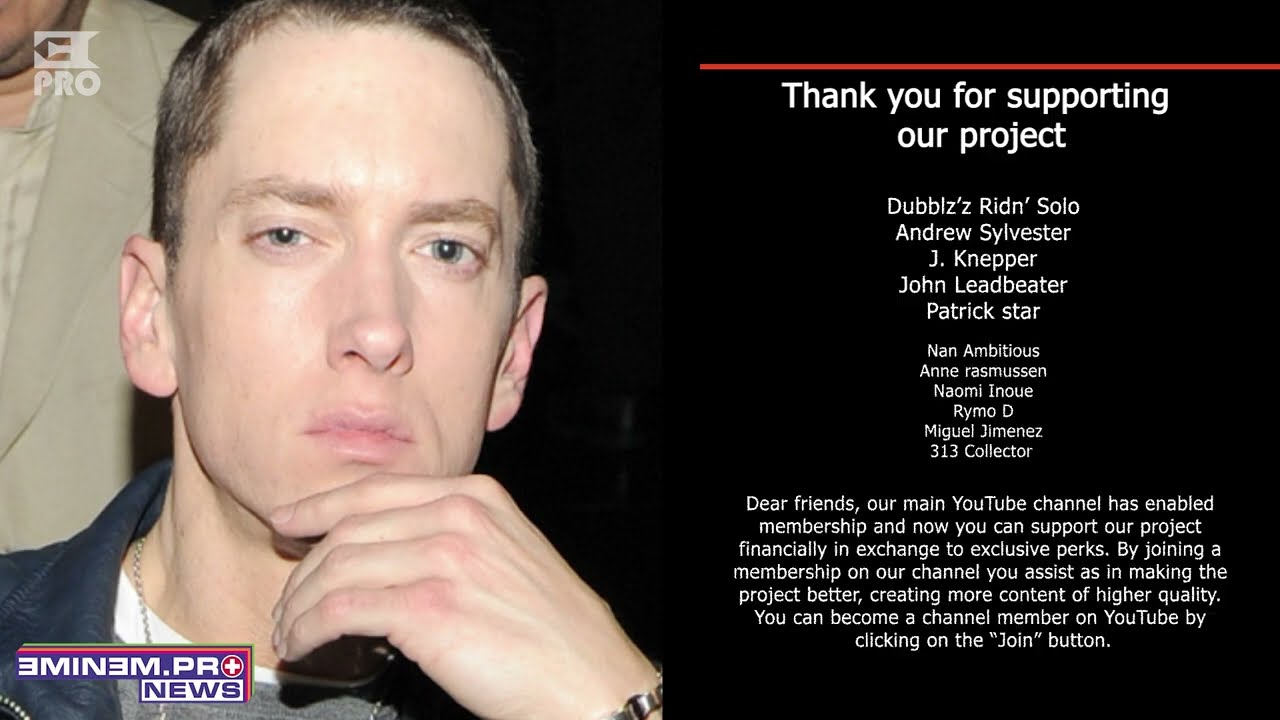In a black background, this poster features a centered image of rapper Eminem on the left side. Eminem, with brown short hair and blue eyes, looks intently into the camera, his expression serious, tinged with sadness. He is dressed in a black down jacket over a grey t-shirt, with his left hand thoughtfully touching his chin. There's a hint of a silver necklace peeking out, and someone barely visible behind him in a tan jacket.

To the right side of the poster, a bold white text with a red bar at the top reads, "Thank you for supporting our project." Below this, a list of names is displayed in white text, recognizing: Andrew Silvester, J. Clapper, John Lickfield, and Patrick Starr, among others in even smaller, less legible text. In the lower left corner of the image, a logo reads, "Eminem.PR News."